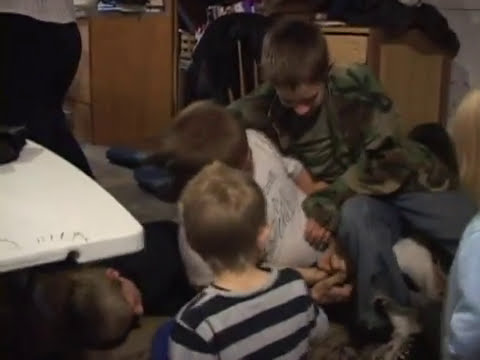The image appears to be a screen grab from a video showing a group of children, likely aged between 8 and 12, engaged in playful roughhousing on what seems to be a carpeted set of stairs inside a house. The setting includes a brown cabinet in the background with clothes on it and a white table next to the children. The scene is somewhat chaotic with several boys tangled together, seemingly wrestling. One of the boys, dressed in a camouflage jacket, green shirt, and jeans, appears to be cradling or restraining another boy in a white shirt while sitting on top of him. Another boy is lying on the ground possibly tired or just resting from the rough play. Additionally, a smaller child in a striped black and gray shirt is watching the action, and a partially visible girl with light blonde hair is cut off on the right side of the image, wearing a light blue top. The photo shows mostly children with blondish-brown hair, and the resolution is quite blurry, reinforcing the impression that it is a video screen grab.